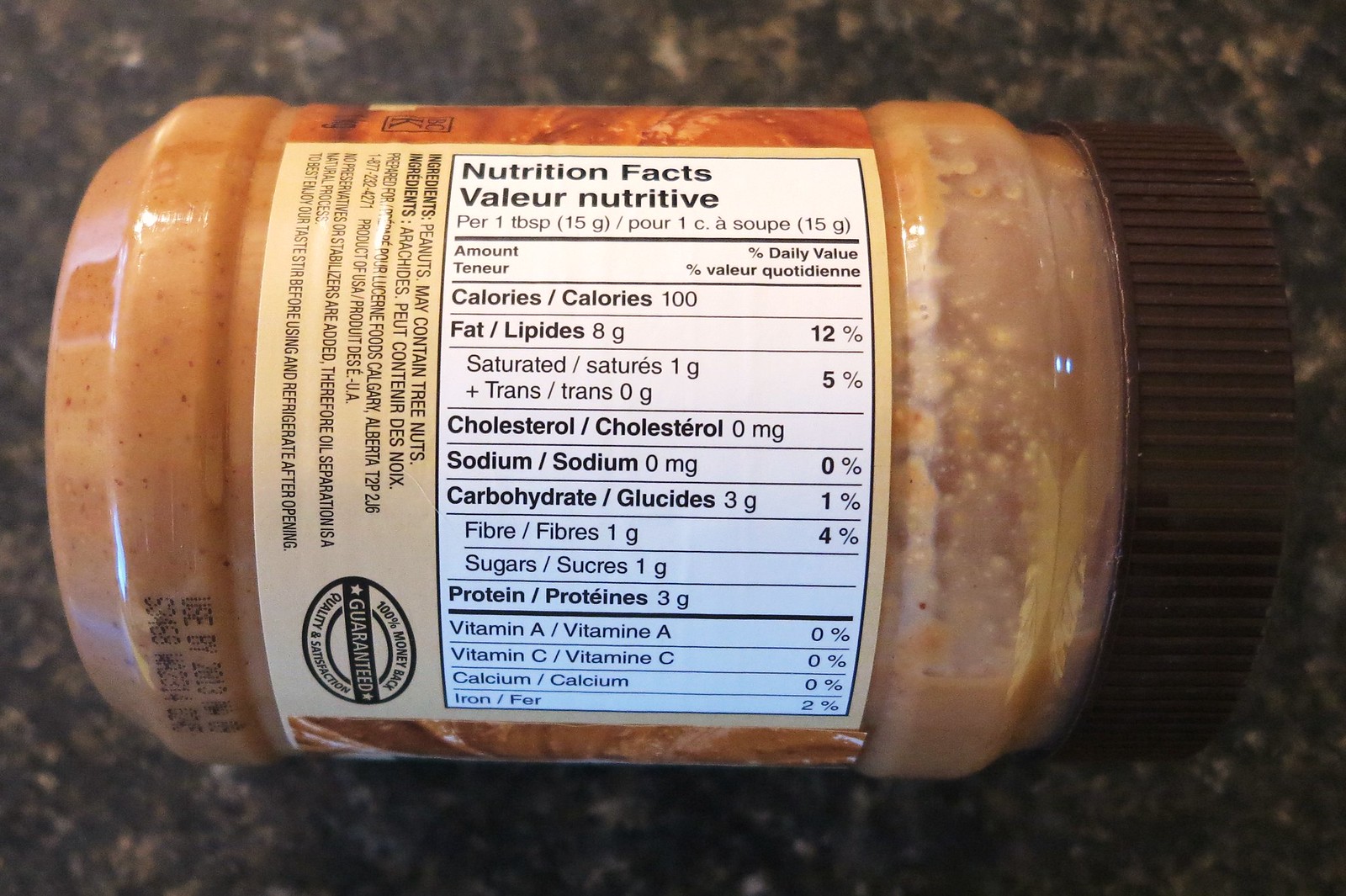This close-up photograph features a jar of natural peanut butter resting on its side on a dark, mottled marble kitchen countertop. The jar has a brown lid and prominently displays its nutritional facts label. Detailed on the label are the serving size, calorie content, fat grams, cholesterol, sodium, carbohydrates, proteins, and vitamins and minerals present in the peanut butter. Beneath the nutritional facts, there is an ingredient label coupled with a logo indicating a money-back guarantee. The expiration date is also visible, providing important information for consumers. Inside the jar, the creamy peanut butter itself can be seen through the transparent container. The clear and detailed layout of the labels offers a comprehensive view of the product's nutritional content and quality assurance.